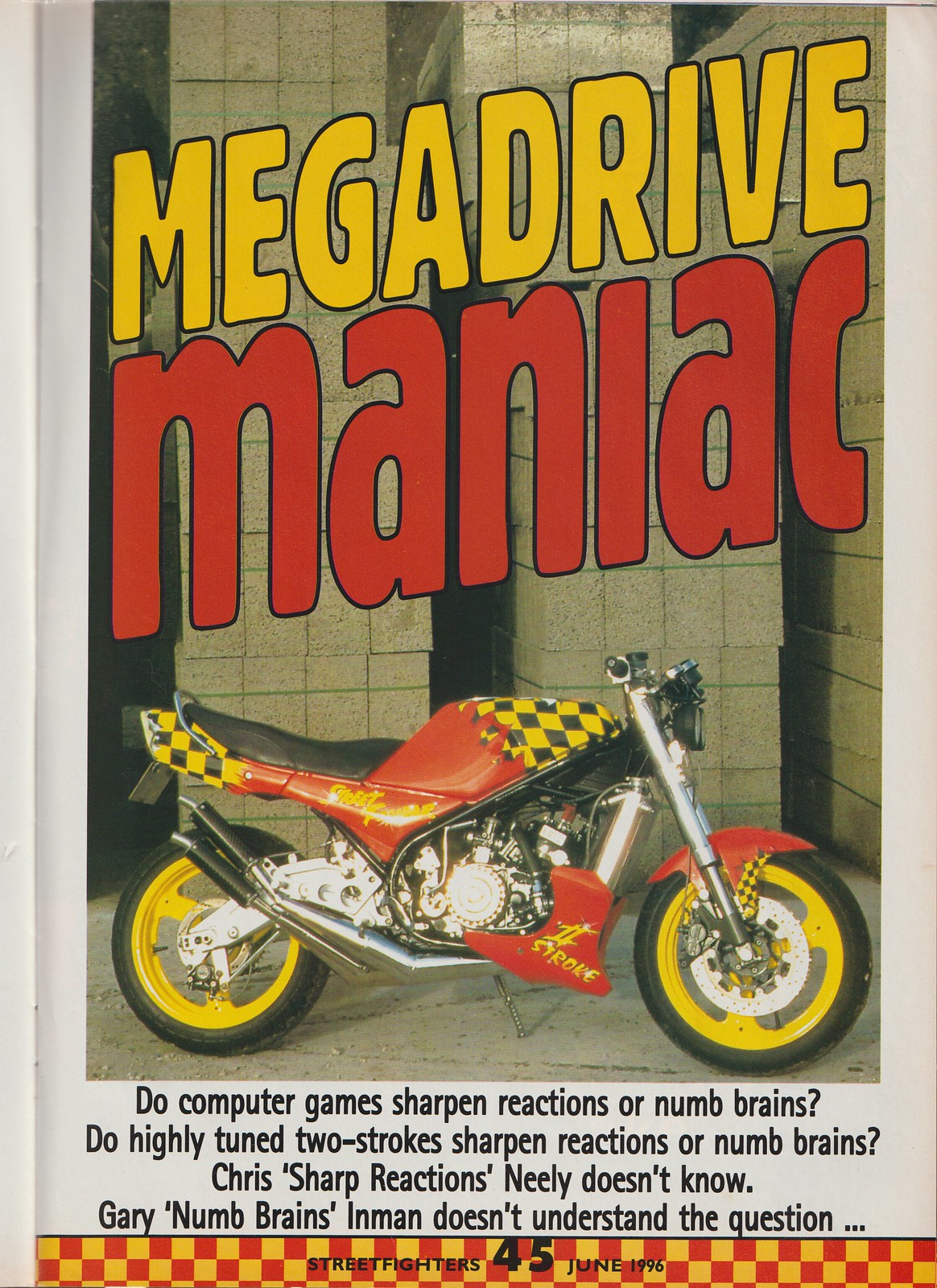This image appears to be an advertisement, possibly extracted from a magazine page, showcasing a vividly colored motorcycle against a gray tile wall. Dominating the top of the ad, the words "Mega Drive" are prominently displayed in bold yellow text. Below that, even larger red text spells out "Maniac." The motorcycle, captured in a side view facing right, is an eye-catching blend of black and yellow with checkerboard detailing and striking red flames. Its wheels are bright yellow, contrasting sharply with the black tires. Below the photograph, there is a section of black text discussing whether computer games or high-tuned two-stroke engines sharpen reactions or numb brains, mentioning individuals named Chris and Gary with differing opinions. The bottom of the ad features a narrow banner with a red and yellow checkerboard pattern, overlaid by the number "45" and the caption "Street Fighters 45 June 1996."